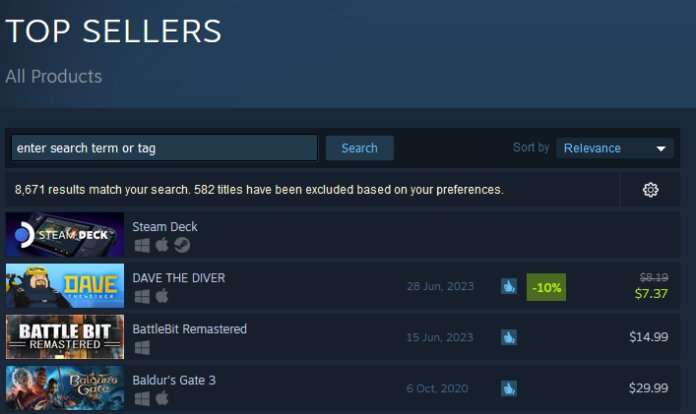The partial image captures a section of a website, most likely a gaming platform such as Steam. In the upper left corner, the text "TOP SELLERS" is prominently displayed in all caps with white font. Directly beneath this is a blue banner that reads "ALL PRODUCTS."

A dark gray banner follows, containing a long rectangular search box with the placeholder text "ENTER SEARCH TERM OR TAG." Adjacent to this is a button labeled "SEARCH." A black space separates this from another section that includes the text "SORT BY" next to a rectangular dropdown box labeled "RELEVANCE," which features a drop-down arrow on its right side.

Below this, to the left, it states, "8,671 results match your search. 582 titles have been excluded based on your preferences." A cog icon is positioned on the far right within a separate box.

Further down, on the left side, "STEAM DECK" is mentioned twice, presumably as a filter or category, accompanied by several icons. Each game listing is associated with a media image. Among these, "Dave the Driver" and "Battle Bit Remastered Baldur's Gate 3" are depicted. "Dave the Diver" is shown with a 10% discount, with the pricing highlighted in green. The STEAM DECK section, however, does not display any pricing information.